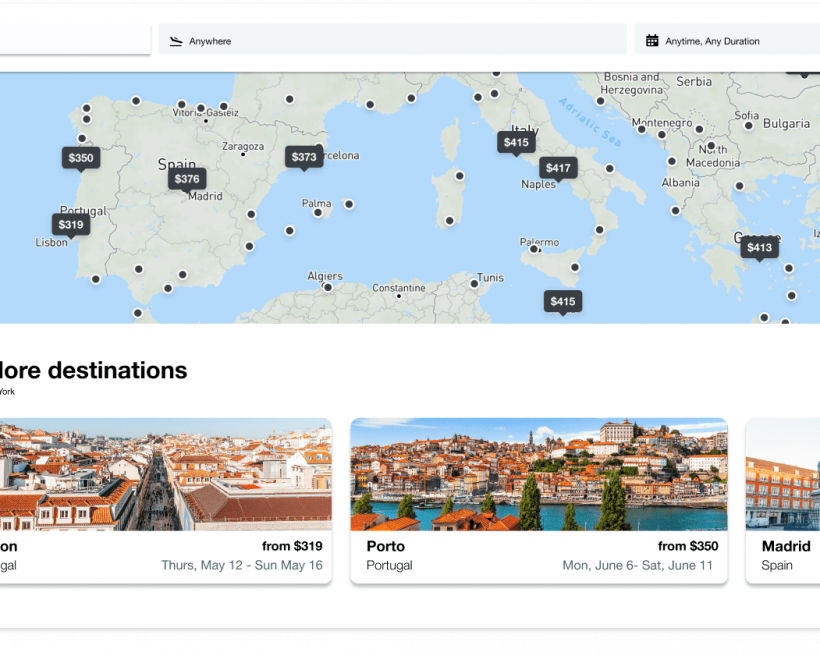This image showcases a detailed map centered around the northern part of the Mediterranean Sea, highlighting several European and African countries with marked destinations and travel prices. The map prominently features Spain, including cities like Madrid ($376), Zaragoza, and Barcelona ($373), as well as the island of Palma. To the west, Portugal is visible, with Lisbon marked at $319 and another generic location at $350.

Moving east, the map displays the border regions of France and Spain, while Italy is detailed with travel prices of $415 to a general location and $417 specifically to Naples, with further dots marking Palermo. The map also shows Greece and the surrounding Balkan countries, including Serbia, Bosnia and Herzegovina, Montenegro, Macedonia, and Albania, with a noted price of $413 for Greece.

In North Africa, Algiers and Constantine in Algeria, as well as Tunis in Tunisia, are labeled. Beneath the map is a section labeled "More Destinations," featuring travel details such as a trip from Lisbon, Portugal from $319 from Thursday, May 12th to Sunday, May 16th, another to Porto, Portugal for $350 from June 6th to June 11th, and travel information for Madrid, Spain, though the details appear to be cut off.